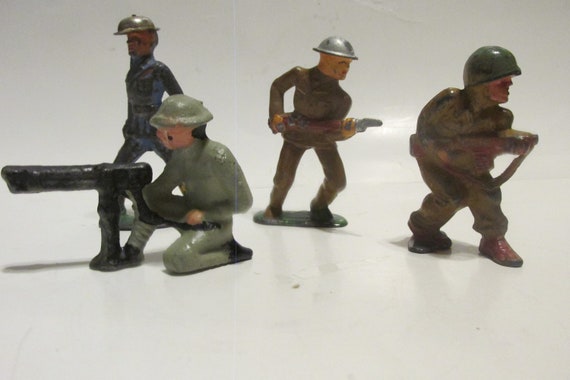In the photograph, four soldier figurines are arranged on a white surface against a white background. These miniature soldiers, possibly from the World War era given their circular Helmets, are detailed but of noticeably poor quality, with one figure showing missing paint and a bluish tinge underneath. Dressed primarily in shades of khaki and green, except for one in blue, the soldiers are posed in various stances—two kneeling, one standing, and one crouched. Three of the figures are armed: two with rifles and one with a large machine gun, positioned on the ground. The figure without a firearm, identifiable by his distinct silver helmet, appears to be the commanding officer, directing the others. The image, showing signs of age with visible wrinkles and lines, captures the figures in dynamic positions indicative of a combat scenario.